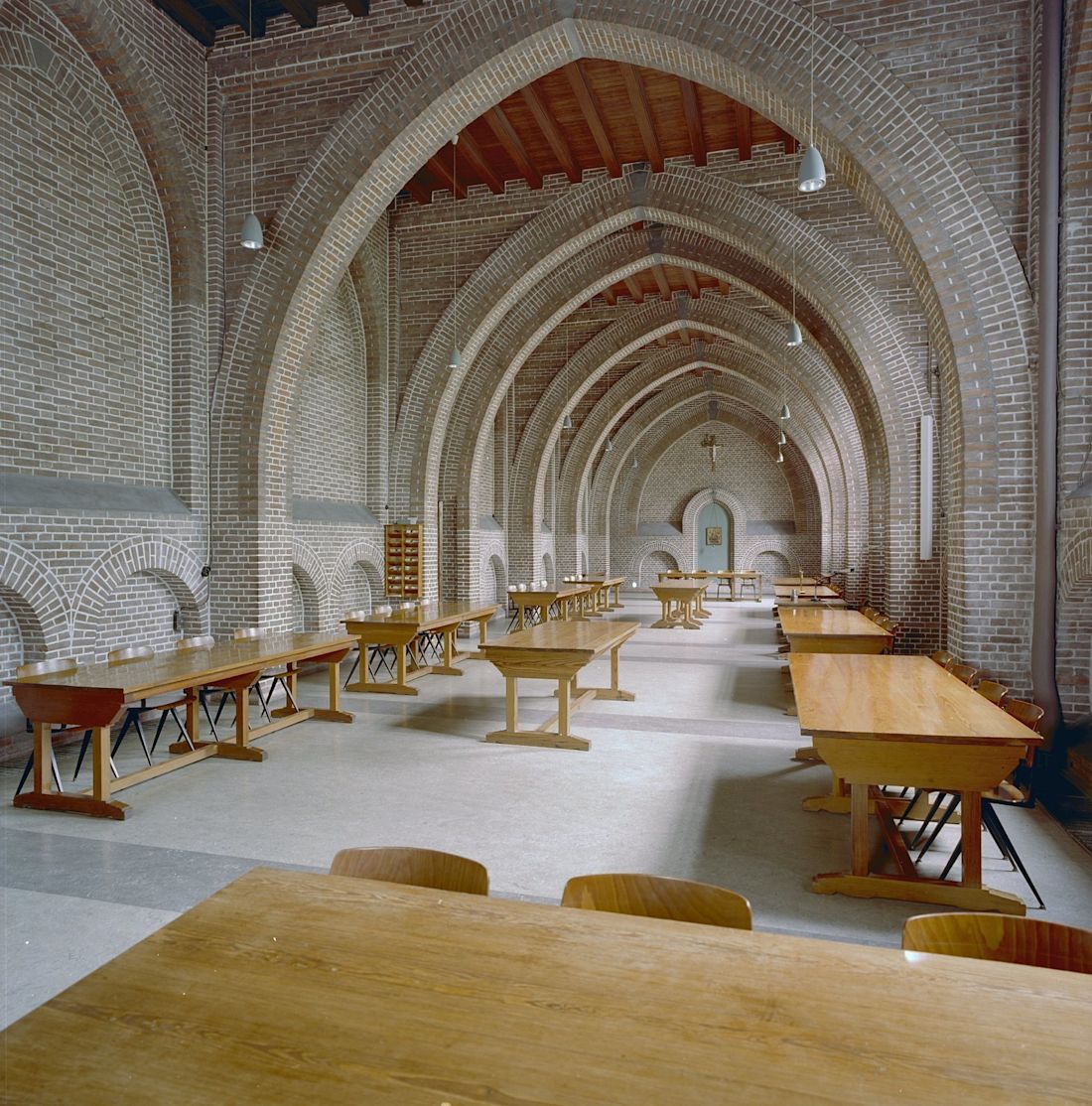This image captures the interior of an old, well-preserved building, likely a dining hall in a college or church setting. The room is expansive, stretching off into the distance with an approximate ceiling height of three stories. The structure boasts high, rounded archways supported by brick columns, revealing a fusion of architectural beauty and historical charm. The brick walls, tinged with a grayish hue, are immaculate, complementing the dark wooden beams and rafters of the ceiling, which also features wooden slats.

The polished gray floor, intersected by darker gray lines at regular intervals, adds a touch of modern upkeep to the ancient ambiance. Arranged throughout the hall are varnished and polished light wood tables and matching chairs, possibly set up for a meeting. In the far distance, a small archway door is visible, adorned with a rectangular sign that remains indistinct due to the distance. This door appears to be the same grayish color as the woodwork. Additionally, hanging lights illuminate the room, enhancing its charm. The structural elegance is completed by a round door with a cross above it, presumably leading to another part of the building, hinting at a religious aspect such as a Catholic school, a church rec room, or a seminary.